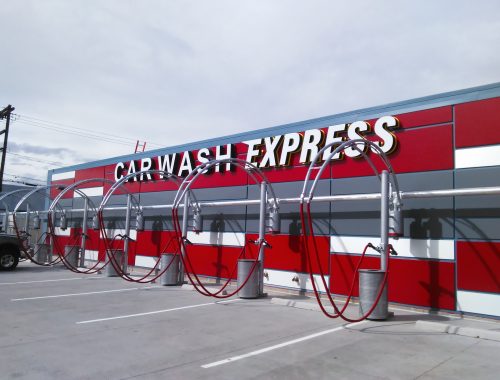The image captures a Car Wash Express building characterized by its red, white, and gray color scheme. The prominent sign at the top of the building reads "CAR WASH EXPRESS" in bold, white capital letters, with the word "Express" slightly italicized against a red background accented by white blocks. The building itself has a pattern resembling a red and white checkerboard on its gray facade. In the foreground, there are five or six parking spaces marked by white lines on light gray pavement, each equipped with red and silver vacuum machines. These vacuums feature red hoses hanging in a swag formation, and cylindrical gray bases. The scene includes a dull gray, overcast sky with a few dispersed clouds and a telephone pole with wires visible at the far left edge of the image. One car is partially visible at the vacuum area in the corner, completing the composition.